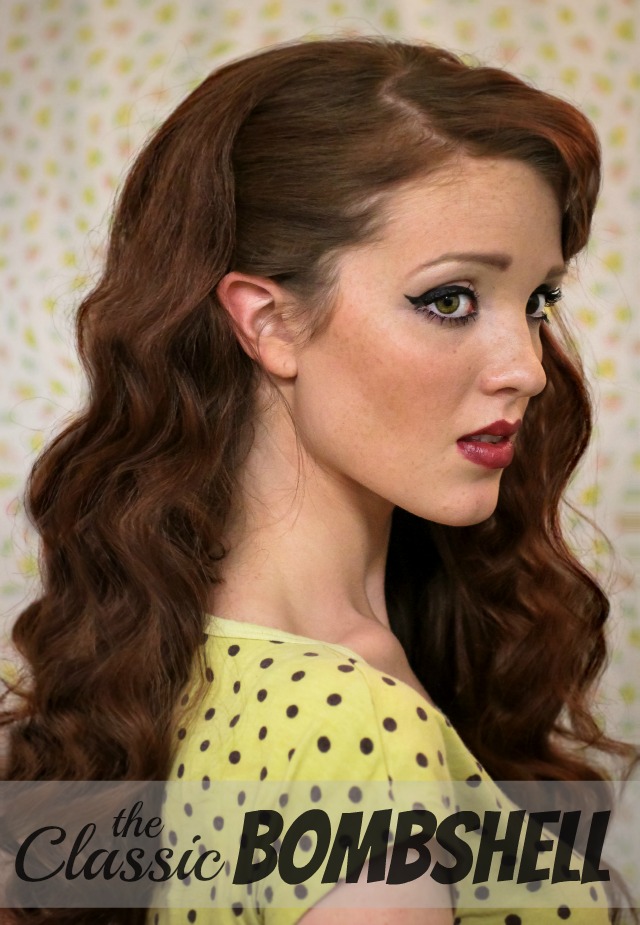In this portrait-oriented image, a young white woman with long, wavy brown hair, parted on the side and lightly pulled back behind her ear, is featured. She stands in front of a cream background decorated with colorful specks in yellow, red, and green. Her head is slightly turned towards the camera, with her striking green eyes looking just past it. She wears heavy, thick eyeliner paired with smudgy under-eye makeup, prominent 80s-style blush, and Clinique Black Honey lipstick. Her outfit is a yellow blouse adorned with black polka dots. At the bottom of the image, the caption reads, "The Classic Bombshell."